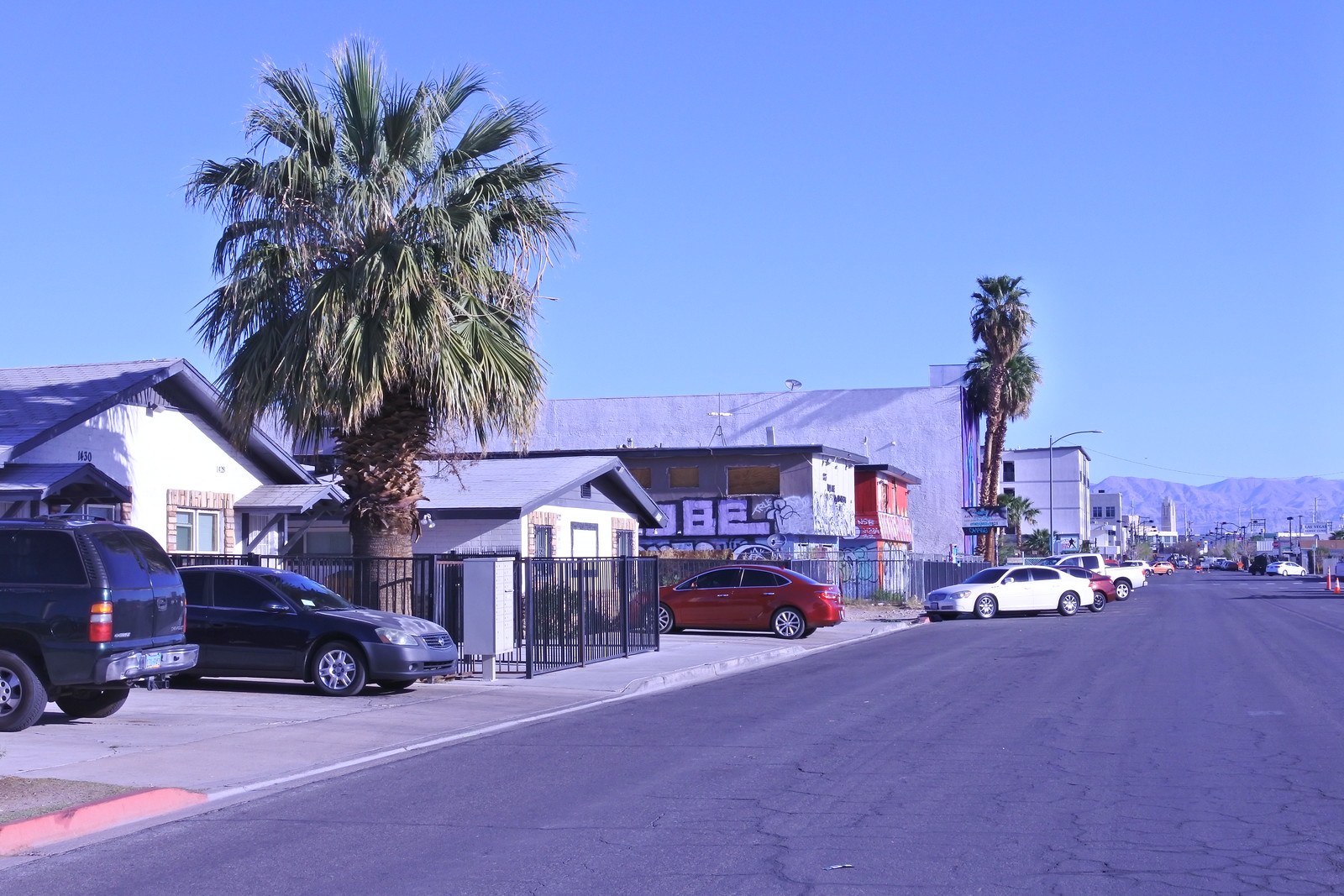The image captures a wide-open, sun-drenched road, likely in an inner-city area in a hot region of America. To the left, there are small bungalows, each with driveways hosting several parked cars. Further back, larger industrial buildings rise, marking a transition from residential to commercial zones. The expansive right side of the road accommodates numerous vehicles parked along its edge. Palm trees punctuate the scene, with one particularly tall specimen prominently situated on the left. In the distant background, a rugged mountainous ridgeline stretches across, contrasting sharply with the flawlessly blue, cloudless sky. The atmosphere is distinctly dry and intensely sunny, reflecting the arid climate.